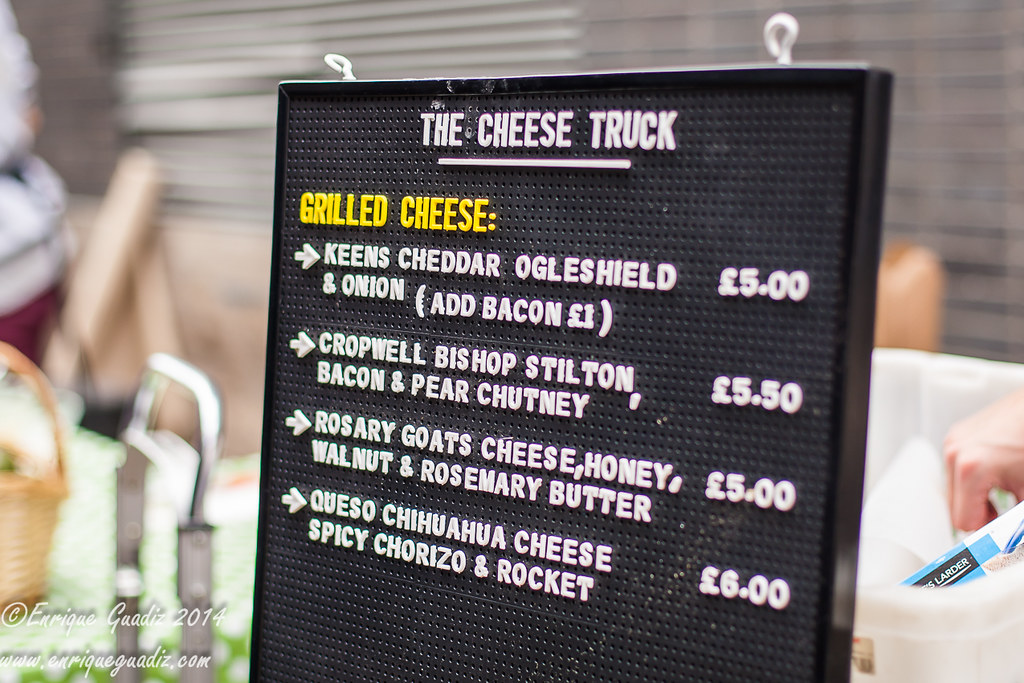The image showcases a detailed, full-color photograph of a pegboard-style menu sign intended for a food truck called "The Cheese Truck." The sign prominently features the menu options, set against a black background with white and yellow letters. It offers various gourmet grilled cheese selections: Keene's Cheddar, Ogleshield, and Onion for £5.00, with an optional bacon addition for £1.00; Cropwell Bishop Stilton, Bacon, and Pear Chutney for £5.50; Rosary Goats Cheese, Honey, Walnut, and Rosemary Butter for £5.00; and Queso Chihuahua Cheese with Spicy Chorizo and Rocket for £6.00. The sign is currently not in use but placed on a counter surrounded by miscellaneous items, including a basket, a white plastic container, and a partially visible person's hand. An inscription at the bottom left corner reads "Enrique Galdez 2014 www.enriquegaldez.com," serving as a watermark, and reinforcing the handcrafted aspect of this gourmet offering.